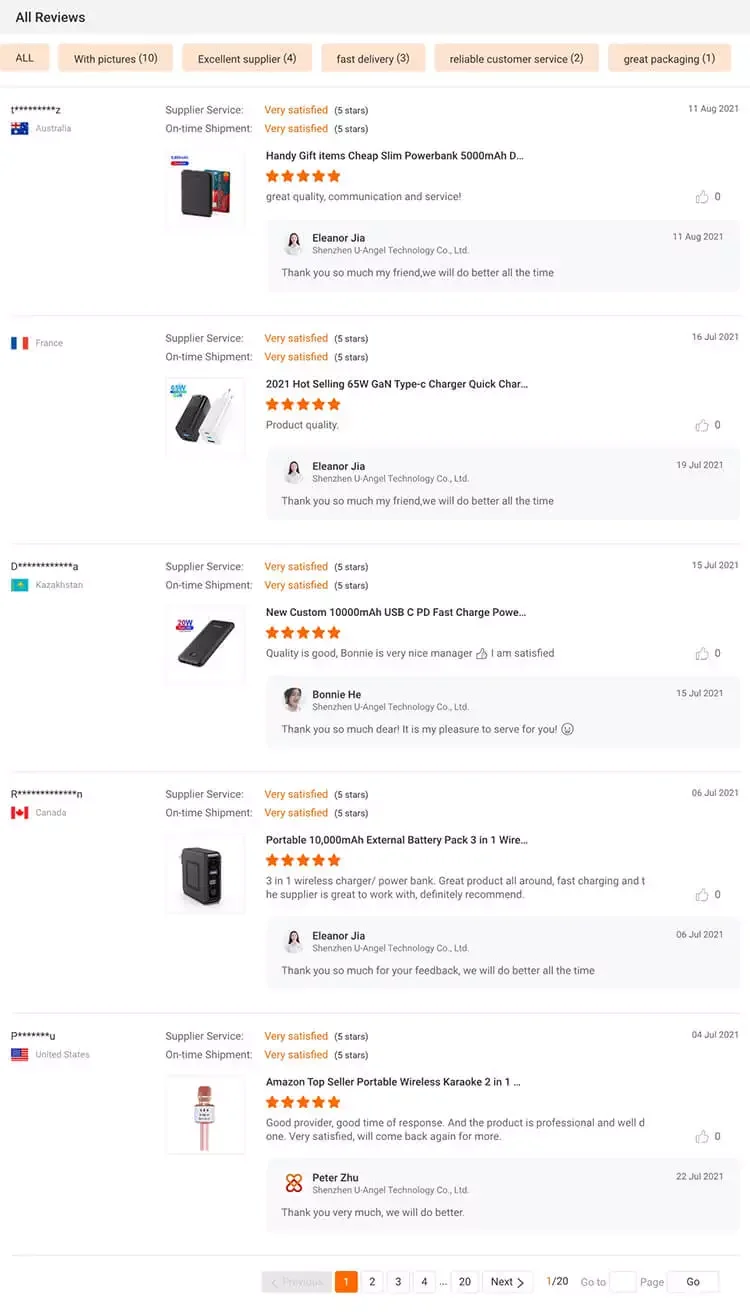The image displays a screen showing a review section titled "All Reviews." At the top of the screen are six filter options: "All," "With Preference," "Some," "Easy Delivery," and two additional options that are not specified but are part of the selection bar. None of these filter options appear to be currently selected.

Below the filter options, there are five distinct items listed, each seemingly sold by different vendors. The items are described as technological products. Each item has a review rating displayed prominently, with all of them showing an impressive five-star rating.

Additionally, the reviews are categorized under two sections: "Very Satisfied" and "Very Dissatisfied," though it is not specified how many belong to each category. The names of the items are mentioned clearly in the reviews, indicating their identity. On the right side of each review, the dates of when these reviews were posted are visible, providing a timeline for each review entry.